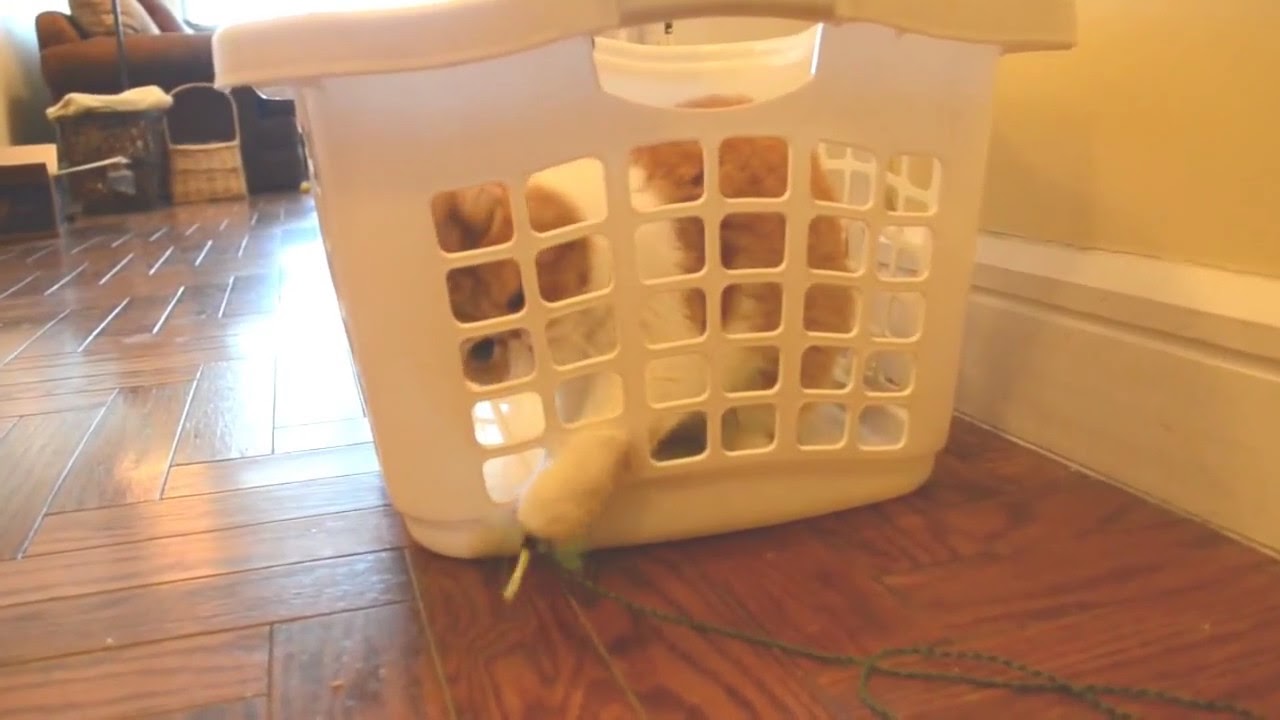The image captures an indoor scene with a white laundry basket positioned on a hardwood floor, surrounded by a warm and cozy environment. Inside the basket, which has a grey handle and patterned grid of holes (about six across and five down), is an orange and white cat. The cat's distinctive pattern features light brown around its head and lower torso, with white on its front shoulders and legs. 

With its left paw (on the right side of the image) extended through the grid, the cat is playfully grabbing at a green shoestring that has a white tip. The shoestring dangles downward towards the hardwood floor. Through the basket's holes, the cat's focused eyes and curious expression are observable, suggesting that it might be eyeing a toy.

The surroundings add a homely touch with a visible strip of white baseboard molding along the base of a yellow-colored wall. The scene also hints at a living area or hallway, as there is mention of sunlight hitting the floor, a chair, a lamp, and possibly a sofa and various baskets in the background. The overall ambiance of the image is warm and inviting, capturing a quintessential moment recognizable to cat owners.